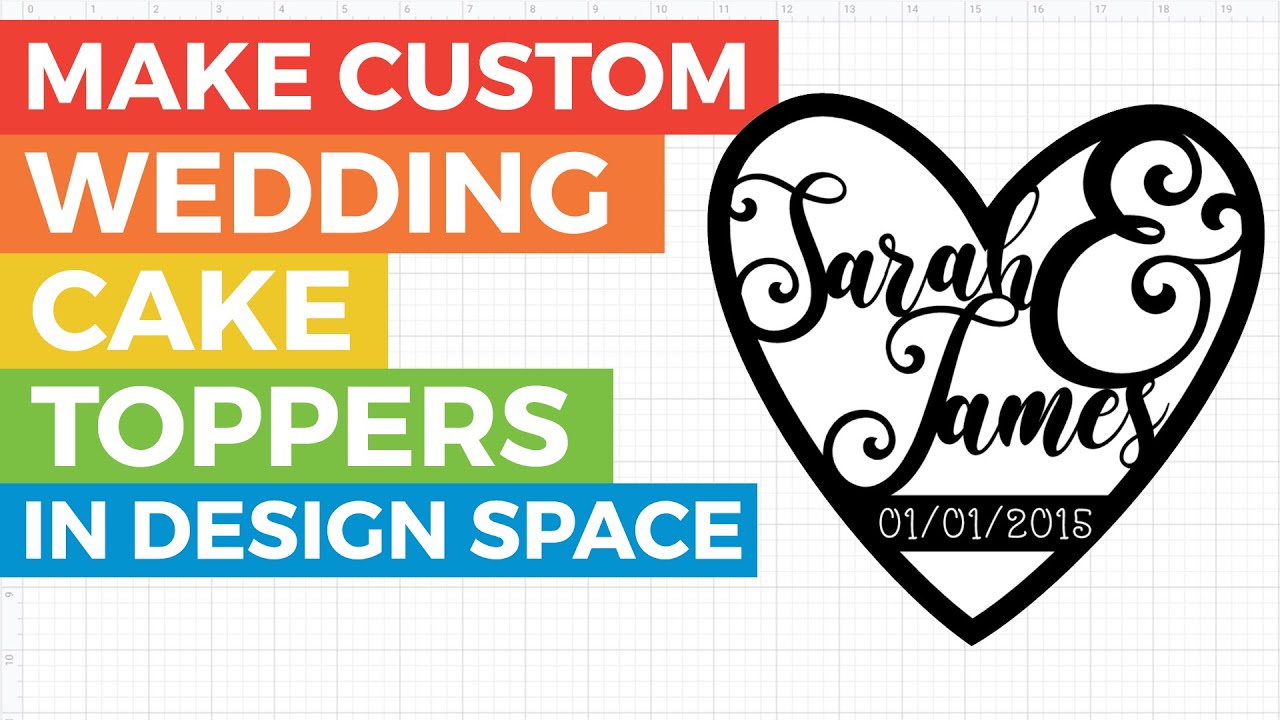This image appears to be a screenshot from a design program with a light gray, graph-paper-like background that is marked from 0 to 19 at the top. On the left side, there are five horizontal rectangles, each filled with a different color: red, orange, yellow, green, and blue. These rectangles contain white, all-caps, sans-serif text that reads, in sequence from top to bottom, "MAKE CUSTOM," "WEDDING," "CAKE," "TOPPERS," and "IN DESIGN SPACE." To the right side of the image, there is a black, unfilled heart that features the names "Sarah Ann James" in cursive black lettering. Below the names, within the heart, there is a small black strip containing the date "01/01/2015" in white font.